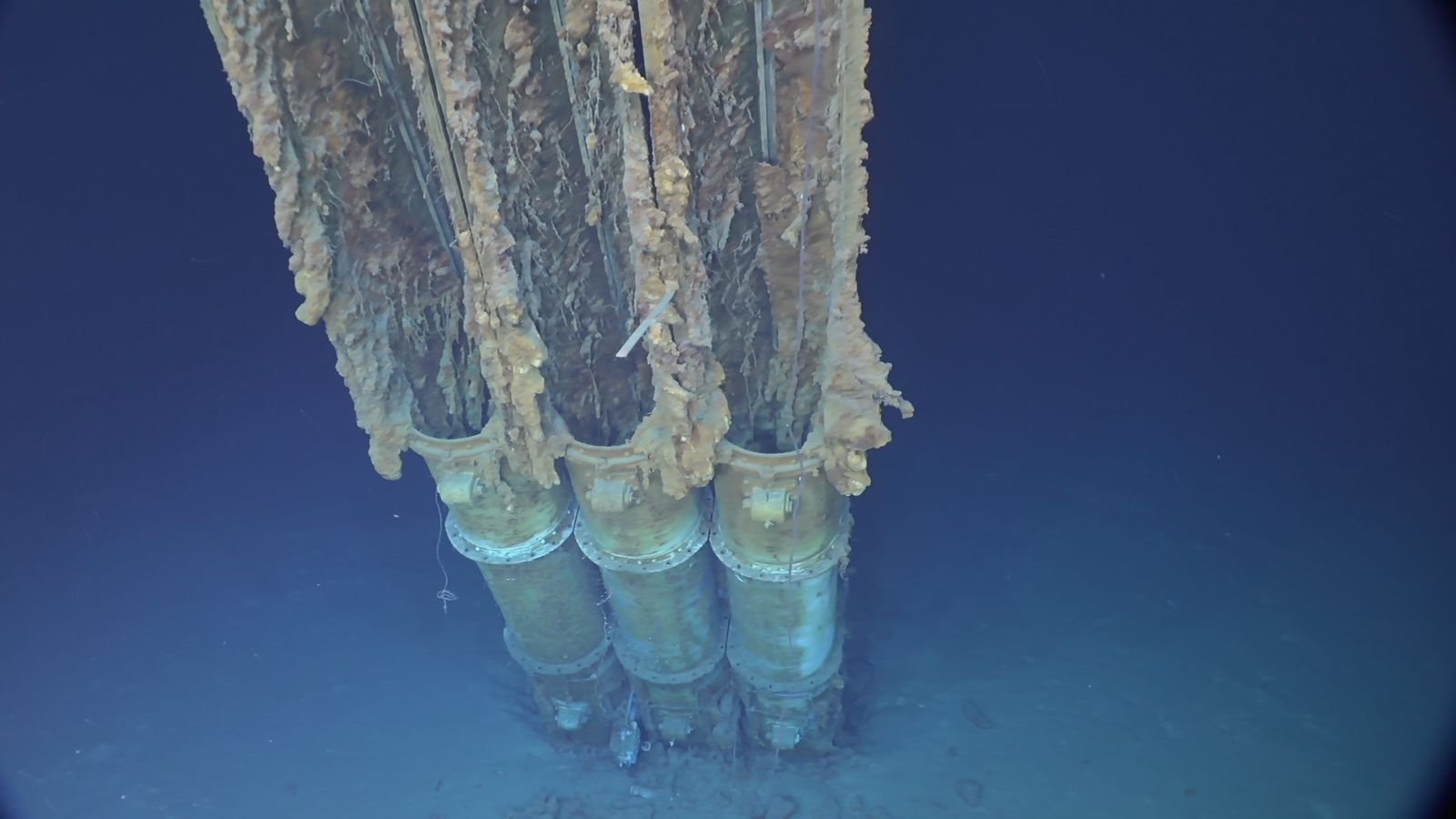The image depicts three items set against a dark blue background. Each item consists of three distinct sections connected by a handle. The bottom section is crafted from see-through plastic, allowing visibility through its transparent surface. Above this, a middle segment is colored in a muted gray tone, offering a subtle contrast. The top section is a combination of brownish hues interspersed with a central white area, adding an intricate detail to the design. Extending from the top, a long, unevenly shaped part emerges, characterized by a dark brown core. This core is enveloped in a textured, brown wrapping that appears wrinkled and irregular, enhancing the unique and tactile nature of the items.